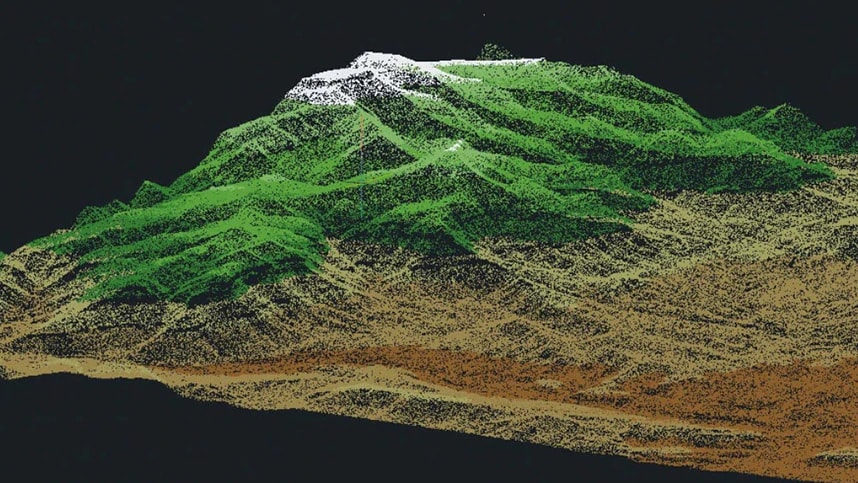This detailed digital rendering showcases the topography of a mountainous terrain, illustrated with a map-like precision. Dominating the black background, the terrain is visually segmented into distinct color zones made up of numerous small dots that create a rich texture. At the peak, the mountain is capped in white, possibly indicating snow-covered summits. Just below the peaks, a swath of forest green suggests dense tree coverage and abundant flora. As the elevation decreases, the colors shift to a brown and beige mid-portion, representing soil and earth. The lowest part is marked by a burnt orange hue, which introduces a unique contrasting strip at the base of the terrain. This computer-generated 3D topographical map, with its detailed ridges and features, gives an impression of what a real mountain might look like in both elevation and composition, highlighted beautifully against its stark black backdrop.